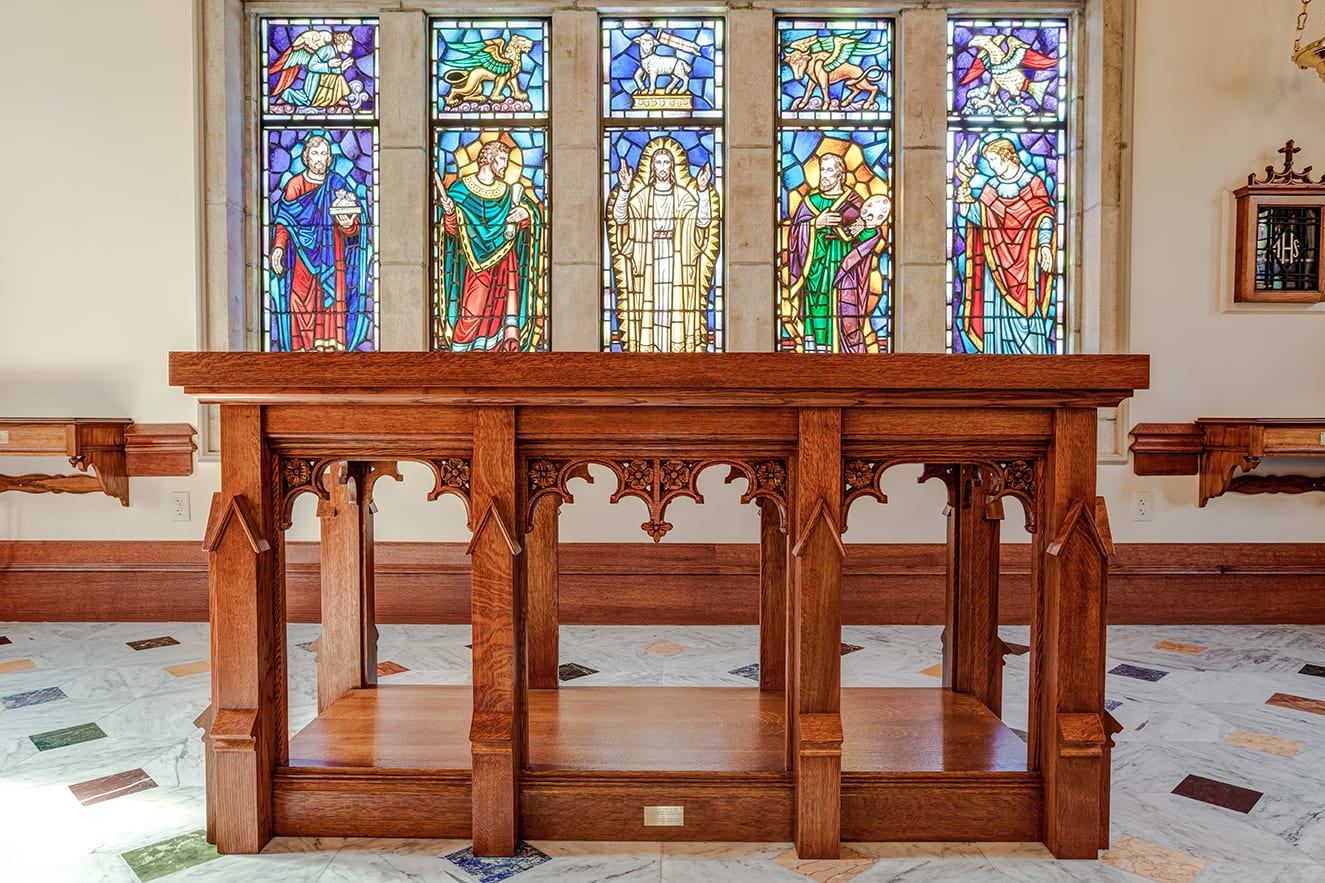This photograph captures the interior of a church, prominently featuring a well-maintained, ornate wooden podium or pulpit with detailed carvings. The pulpit stands on a distinctive white tiled floor patterned with colorful squares in hues of blue, green, yellow, and red. 

In the background, the church's white walls hold five large, vibrant stained glass windows. The central window showcases a revered image of Jesus Christ with a lamb above him, while saints are depicted in the two windows on each side. At the top of each window are smaller, intricate sections representing different figures: a man, a lion, a bird, and another man kneeling down. 

Flanking the windows, wooden shelves are attached to the wall; on the right side, a small cabinet adorned with a cross sits above the shelving. Additionally, a hanging light fixture is visible in the top right corner, adding to the intricate details of the space. This richly decorated scene beautifully captures the solemn and sacred ambiance of the church interior.